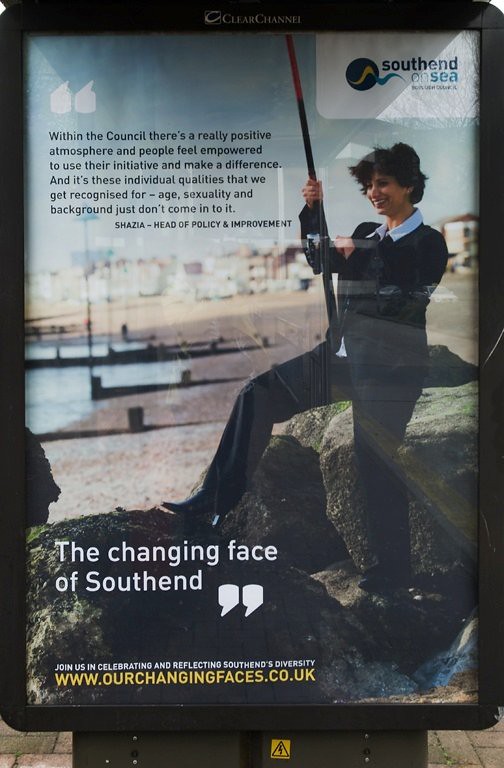The image depicts a billboard advertisement featuring a smiling woman, likely in the UK, associated with the campaign "The Changing Face of Southend" from www.ourchangingfaces.co.uk. The woman, dressed in a white collared shirt and dark outerwear, appears to be fishing, either standing on a rock or off a dock, with her foot placed firmly on some rocks, suggesting a beach setting. The advertisement prominently displays a quote from Shazia, Head of Policy and Improvement, stating, "Within the council, there's a really positive atmosphere, and people feel empowered to use their initiative and make a difference. It's these individual qualities that we recognize; age, sexuality, and background just don't come into it." This campaign aims to celebrate and reflect Southend's diversity, as highlighted by the slogan at the bottom of the billboard.